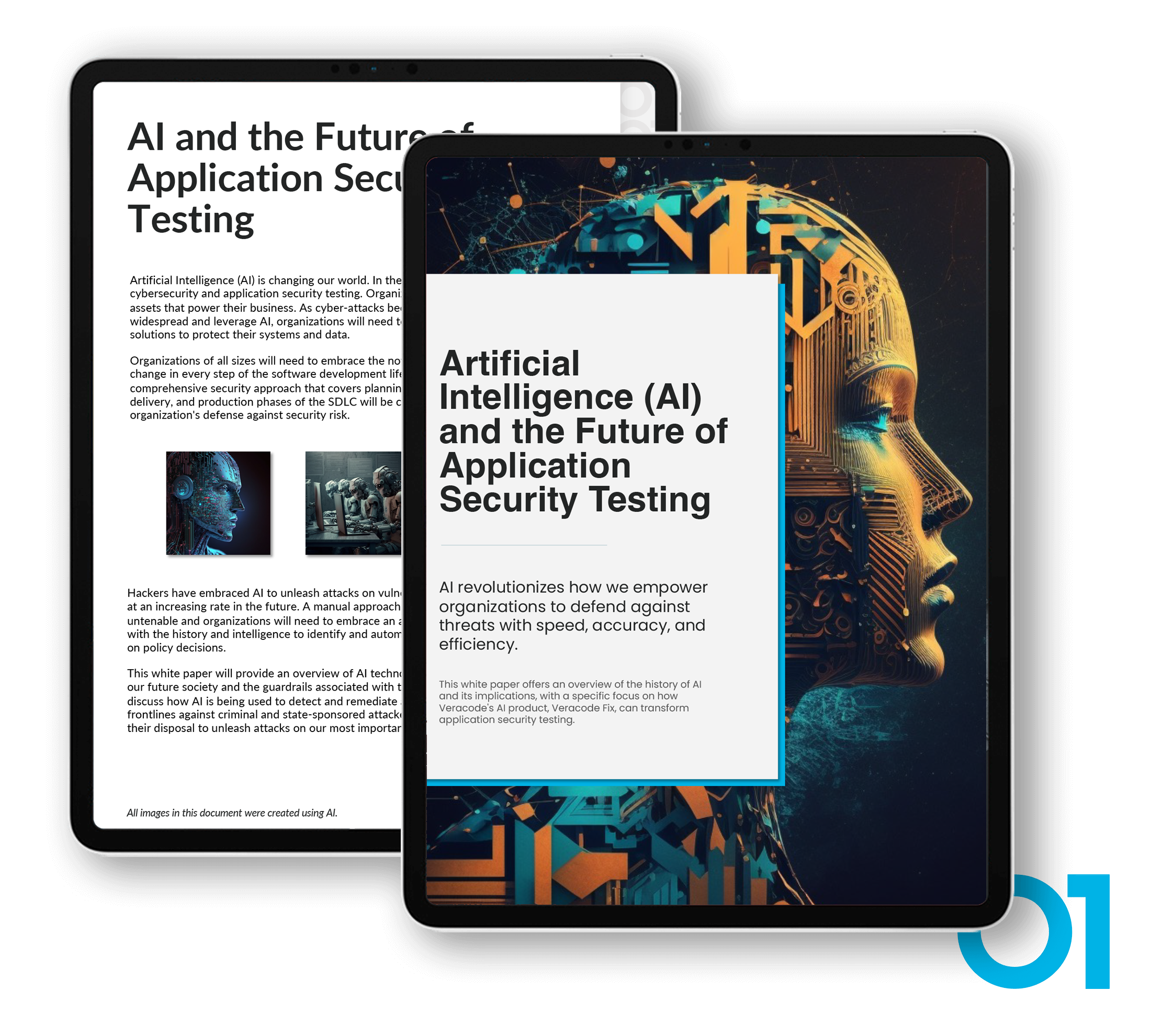The image features two tablet screens, with one slightly overlapping the other, both displaying content related to artificial intelligence. The tablet in the foreground highlights an article titled "Artificial Intelligence and the Future of Application Security Testing." Below the title, the article states, "AI revolutionizes how we empower organizations to defend against threats with speed, accuracy, and efficiency." This screen has a dark blue background and features an artistic depiction of a robotic face looking to the right, embellished with gears and mechanical elements in shades of blue and hints of orange or gold.

The tablet in the background, partially obscured by the foreground tablet, also discusses AI, but its text is mostly unreadable due to the overlap. However, it is evident that it relates to similar themes of future applications and security testing. This background tablet has a white background with dark blue or black print and also features an AI robotic face imagery. Notably, at the bottom right corner of the foreground tablet, the number "01" is visible, suggesting it may be the first page of a multiple-page document.